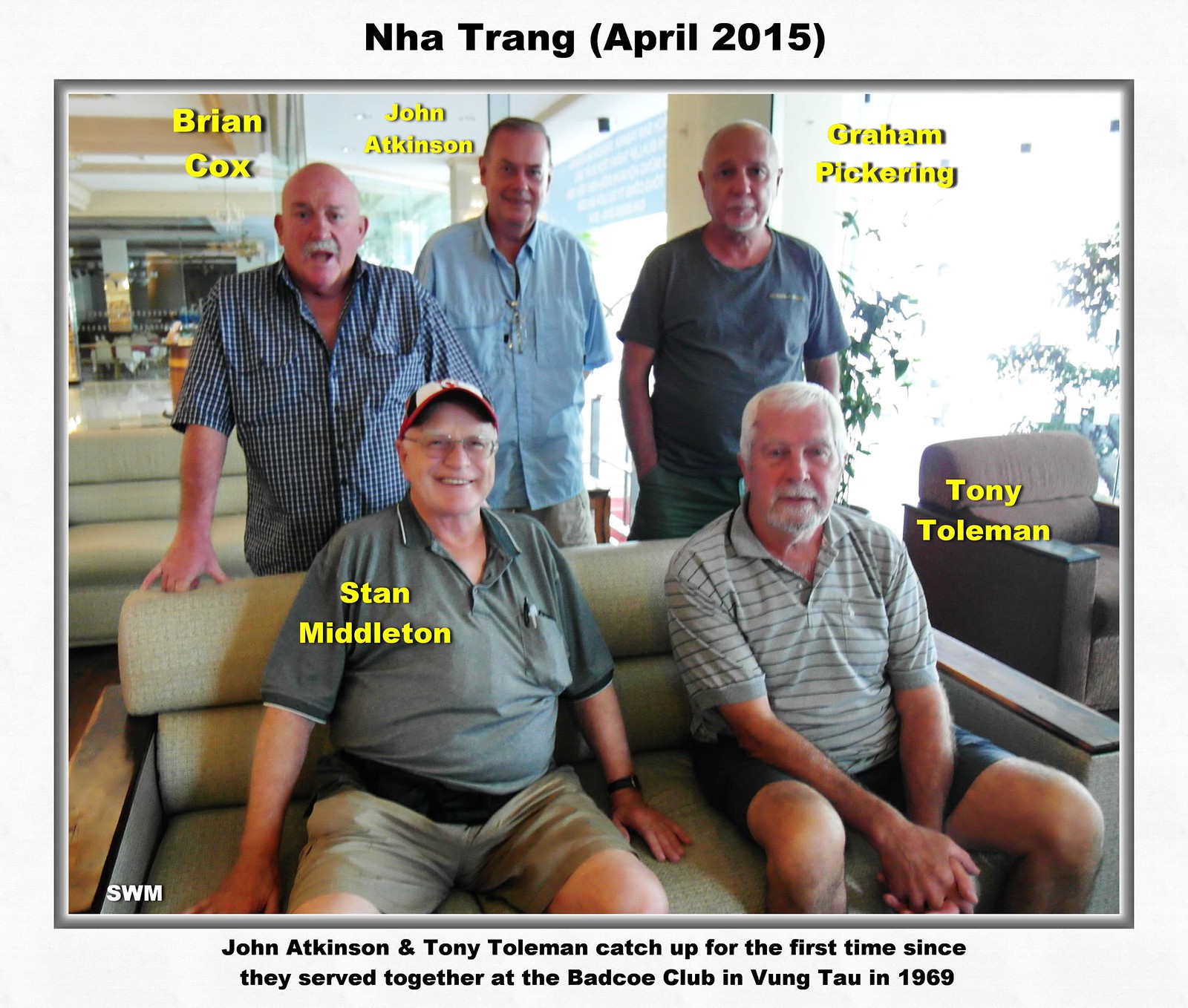This is a detailed reunion photograph taken in April 2015, captioned at the top with "Nga Trang, April 2015." The image features five elderly men, who appear to be Vietnam veterans, arranged with three standing behind two seated on a love seat. The men are labeled from left to right: Brian Cox, John Atkinson, and Graham Pickering standing in the back, while Stan Middleton and Tony Tolman are seated in the front, with Stan on the left wearing a baseball cap. The text at the bottom states in bold Arial font, "John Atkinson and Tony Tolman catch up for the first time since they served together at the Bad Co. Club in Vung Tau in 1969." Additionally, the initials "SWM" are printed in white in the bottom left corner. All men have whitish or grayish hair, with varying degrees of baldness, and are dressed casually in a mixture of collared shirts and t-shirts, suggesting a relaxed reunion environment, possibly in a daylight-lit hotel lobby.